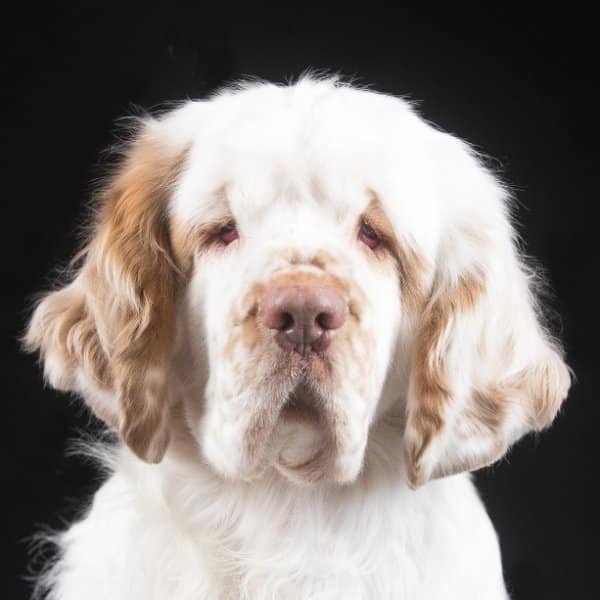This is a high-quality color photo of a large Spaniel-type dog with longer, curly fur, set against a black background. The dog, which has a predominantly white coat, is facing the camera with an attentive yet serene expression. Its left ear is primarily brown with a touch of white at the bottom, while the right ear is mostly white with brownish-orange splotches. The dog's eyes are dark, almost appearing black, with a hint of reddish and pink coloring beneath them, giving a slightly sleepy or aged appearance despite the absence of gray hair. The dog has notable facial features including long jowls and a large pink nose surrounded by brown and orange fur. Brown markings are also visible above and around the eyes, as well as on the snout. The edges of its mouth are pink and slightly open. The overall mature and dignified demeanor of the dog is highlighted by its clear and focused gaze directly at the camera. The simplicity of the black background emphasizes the dog's detailed and varied coloring.